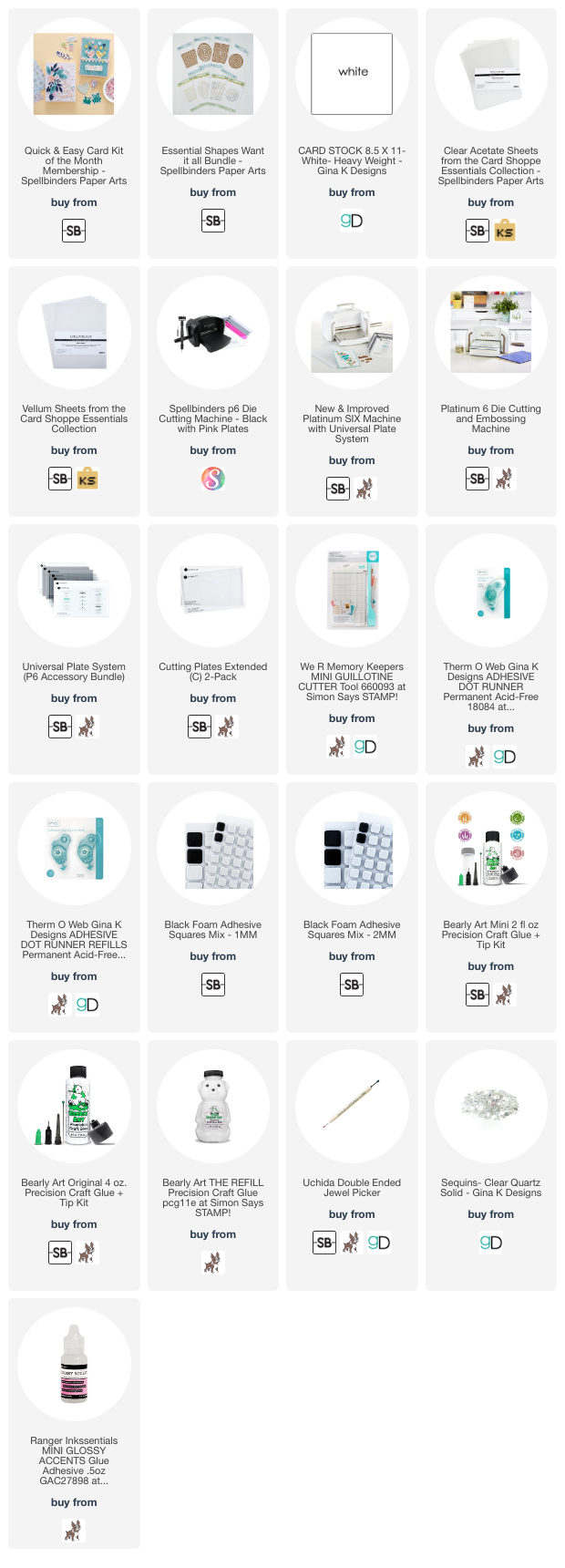The image is a vertically oriented screenshot, likely from a webpage, showcasing a grid of purchasable items. The grid comprises five columns and six rows, with a total of 21 items, including a solitary item placed in the bottom-left corner. Each item is set against a gray background, separated by thin white dividing lines, and bordered by a white edge.

The items depicted are random everyday objects, though their fine details and descriptions are indistinguishable due to their small size. Examples of the items include: 

1. An arts and crafts set in the top-left corner.
2. A piece of paper featuring a cookie design in the second position.
3. An empty honey jar shaped like a bear, positioned slightly to the right.
4. A selection of cleaning supplies.
5. An empty bottle in the lower left, resembling a Gatorade bottle.

The grid showcases a variety of miscellaneous objects, each distinct in shape and design.